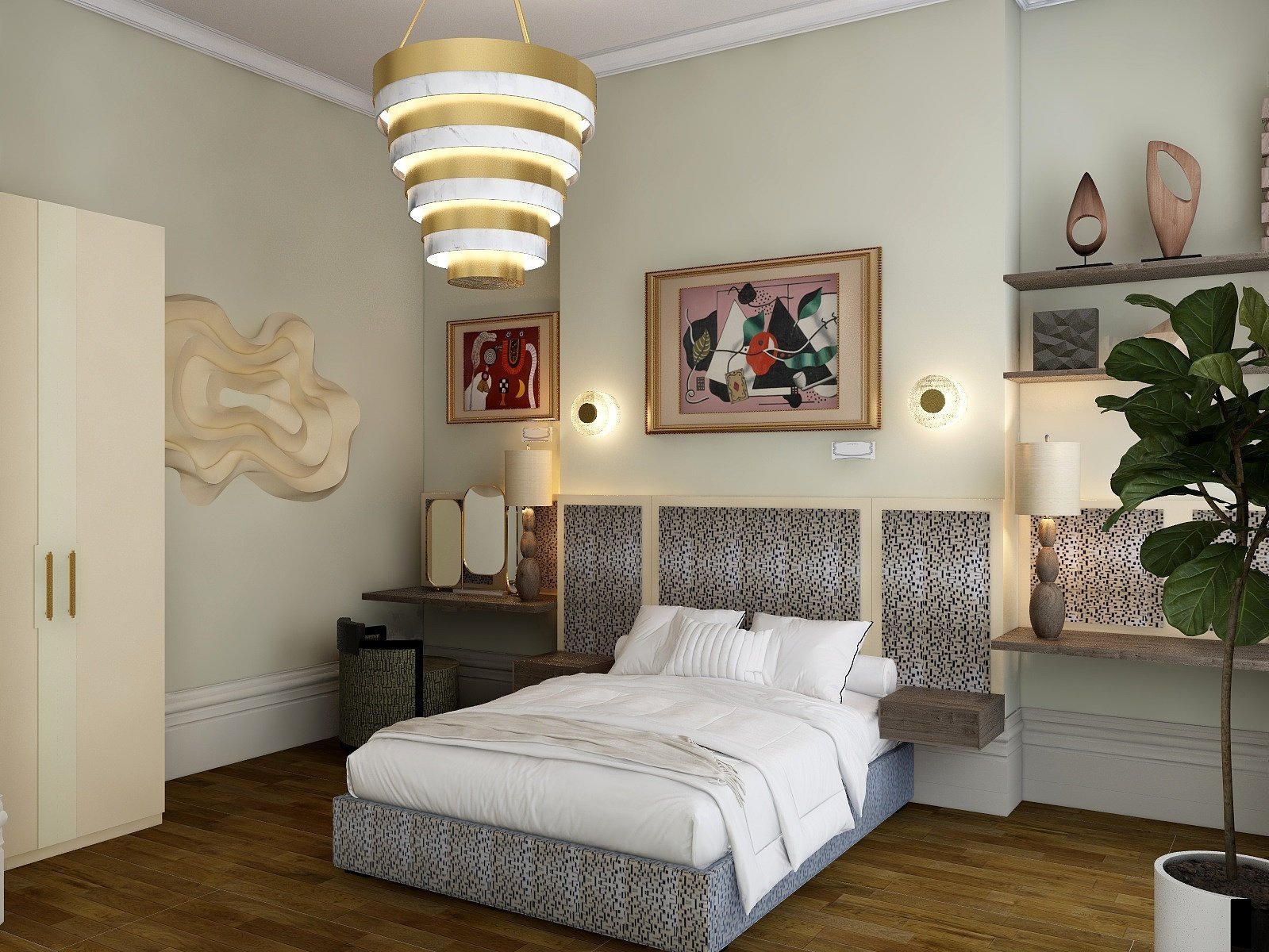This is an indoor photograph set in a modern bedroom with off-white walls and a pure white ceiling. The room features bright white trim, crown molding, and baseboards. Dominating the center of the room is a queen-sized bed with a white bedspread turned down neatly. The bed is adorned with three white pillows and a small pillow arranged in a neat formation against a vibrant blue headboard with a floral print, which coordinates with the base or the box spring of the bed. 

Floating night tables flank either side of the bed, with small lamps perched on top. Above the bed hangs a prominent abstract painting featuring various shapes, housed in a gold frame. To the left of this piece of art is a smaller, similarly framed painting. The walls have a swirly, wavy design interspersed with decorative black and white pattern pads, enhancing the room's style.

On the right side of the image, there are floating shelves displaying an assortment of sculptures, abstract art pieces, and a lamp. A tall potted plant in a white pot stands next to these shelves, adding a touch of greenery. On the far left of the image, there is a compact vanity area positioned near a tall wardrobe unit and a mirror. Completing the scene is an ornate, gold and white layered light fixture that hangs from the ceiling, adding a final touch of elegance to this modern, meticulously decorated, and furnished bedroom.